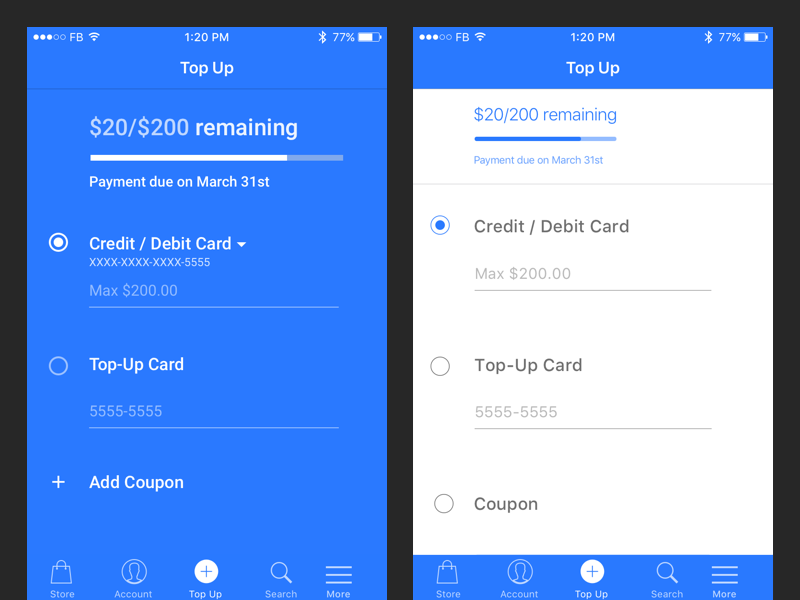This image showcases two smartphone screenshots placed side-by-side against a black background. The photograph itself is square-shaped, and the screenshots are separated by a gray border that blends into the surrounding black border.

**Left Screenshot:**
The left screenshot displays a blue screen with white text and icons at the top. On the status bar, it shows the time "1:20 PM," a full Wi-Fi connection icon, the letters "FB," and three white dots followed by two empty dots. Additionally, there is a Bluetooth signal indicator and a battery icon showing 77% charge. Below the status bar, the main content area features a dark blue background with white text indicating "20 out of 200 remaining dollars" and a payment due date of "March 31st." Below this, there are radio buttons with options for "Credit/Debit Card" or "Top-up Card," with the former being selected. There is an "Add Coupon" button to the right of these options and several items listed at the bottom.

**Right Screenshot:**
The right screenshot has a blue header labeled "Top-up," with the rest of the screen displaying a white background. The information mirrors the left screenshot but features an inverted color scheme. The radio button options and text are black instead of white, and the selected radio button for "Credit/Debit Card" is now blue. At the bottom of the screen, there are icons labeled "Store," "Account," "Top-up," "Search," and "More."

Overall, the image provides a comparative view of two similar screens with slightly different color schemes and layouts, likely from a financial app or service.